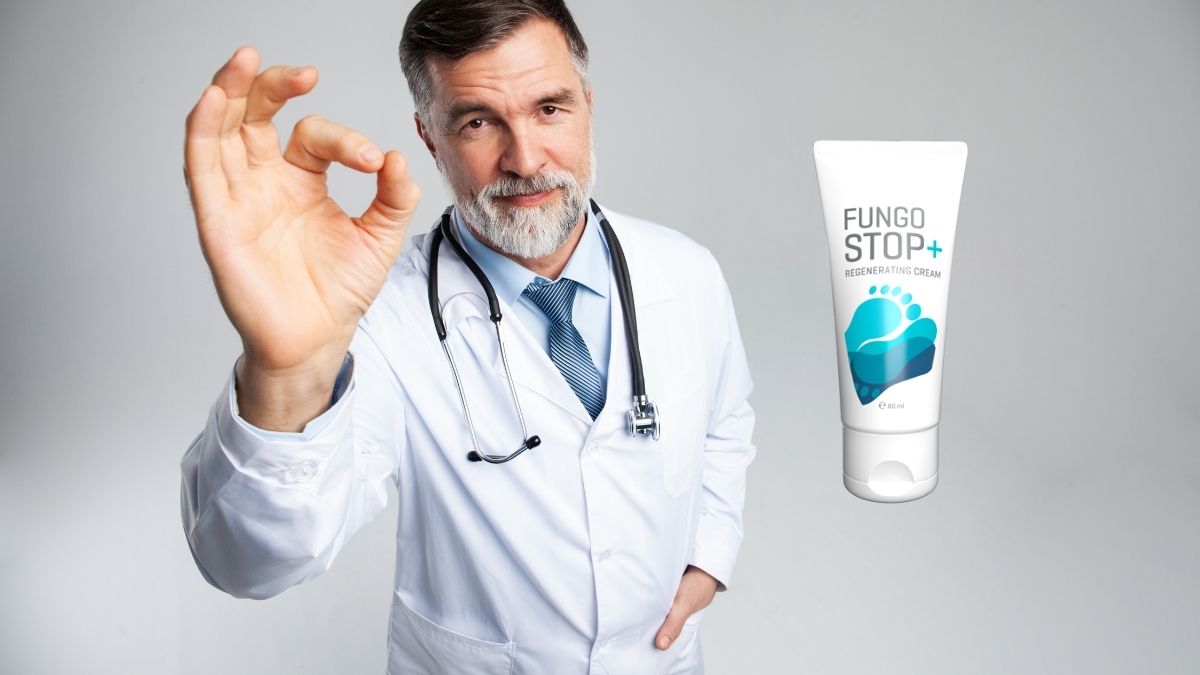The image portrays a distinguished doctor standing against a light gray backdrop with slight shading in the upper left. He is attired in a white coat over a blue button-down shirt and a neatly tied blue tie, with a stethoscope casually draped around his neck. The doctor, with dark hair flecked with gray at the sides and a salt-and-pepper beard and mustache, exudes an air of professionalism. He stands confidently, one hand in his pocket, while his right hand makes the universally understood 'OK' gesture, emphasizing his endorsement. His right hand is positioned close to the camera, creating a dramatic foreshortening effect. Just to his left, prominently featured, is a tube of Fungostop Plus Regenerative Cream. The white tube, marked with turquoise blue graphics and illustrations of two footprints, clearly indicates its purpose—to treat fungal infections of the feet. The overall composition of the image, with its clean lines and clear messaging, strongly suggests that this is an advertisement for the Fungostop Plus product, reinforced by the professional endorsement of the doctor.